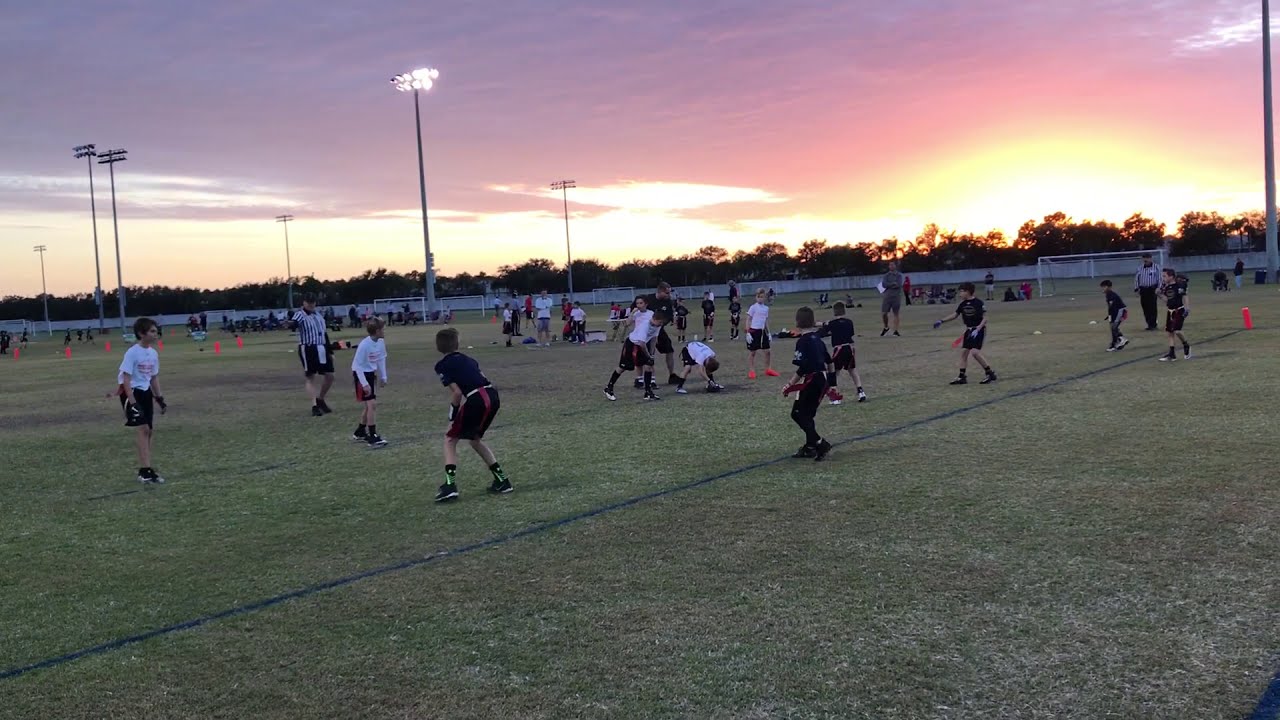In a sprawling, multi-use sports field at dusk, a group of young kids is engaged in a lively flag football practice. The scene is characterized by a vibrant sunset, with shades of pink, orange, and red painting the sky, just as the large overhead lights are about to switch on. The teams are lined up, with one side wearing black jerseys, shorts, and shoes, while their opponents sport white jerseys and black shorts. The kids, appearing to be part of a peewee league, are poised in various energetic stances, ready for action. In the distance, referees and coaches are visible, guiding the young athletes through their drills. Several soccer goals are scattered around the edges of the field, hinting at its multi-use nature. A fence runs along the perimeter, beyond which trees outline the horizon, completing the picturesque setting. There are a few spectators in the background, watching the kids play under the glowing hues of the setting sun.